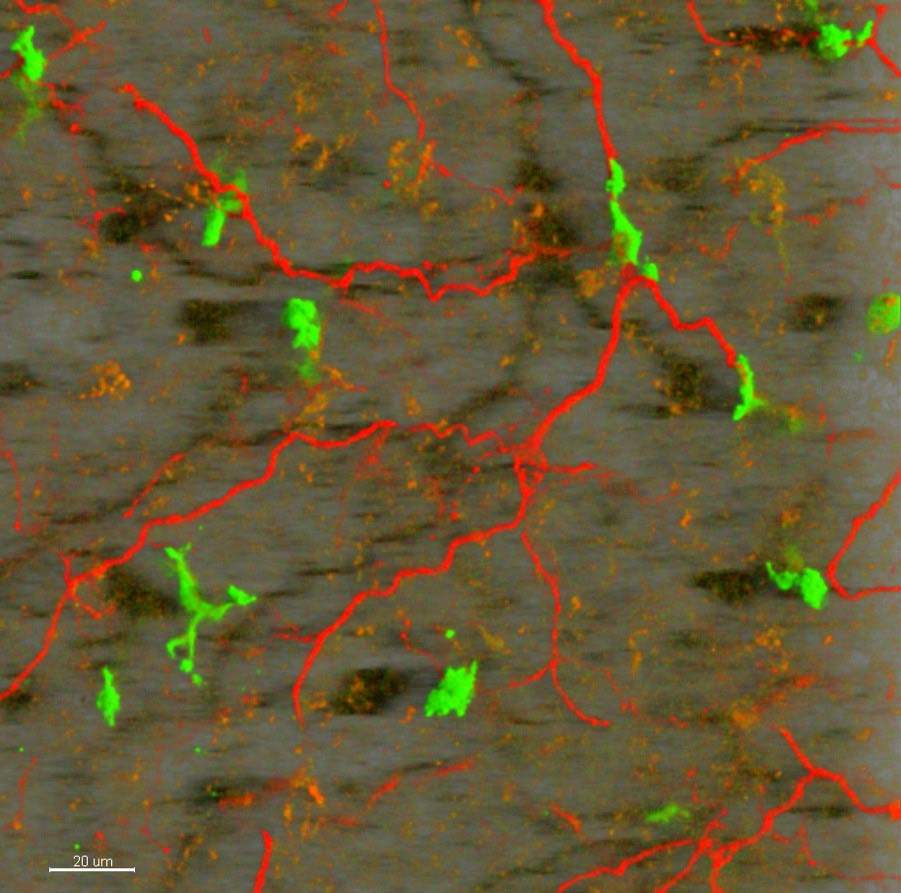This microscopic image features a complex network of vibrant red, lightning-like jagged lines, which seem to be interconnected by bright neon green splotches. The vivid red lines appear to descend across a primarily plain gray background, interspersed with mottled taupe and brown hues reminiscent of a granite countertop. Among these intense colors, there are also blurry orange splotches adding to the intricate scene. Shadows of the red lines can be seen in the background, creating depth. In the lower-left corner, the image includes a scale bar marked "20 UM," indicating a measurement in micrometers for reference. The image is square in shape, capturing a striking, almost surreal view suggestive of biological inscriptions at a micro level.